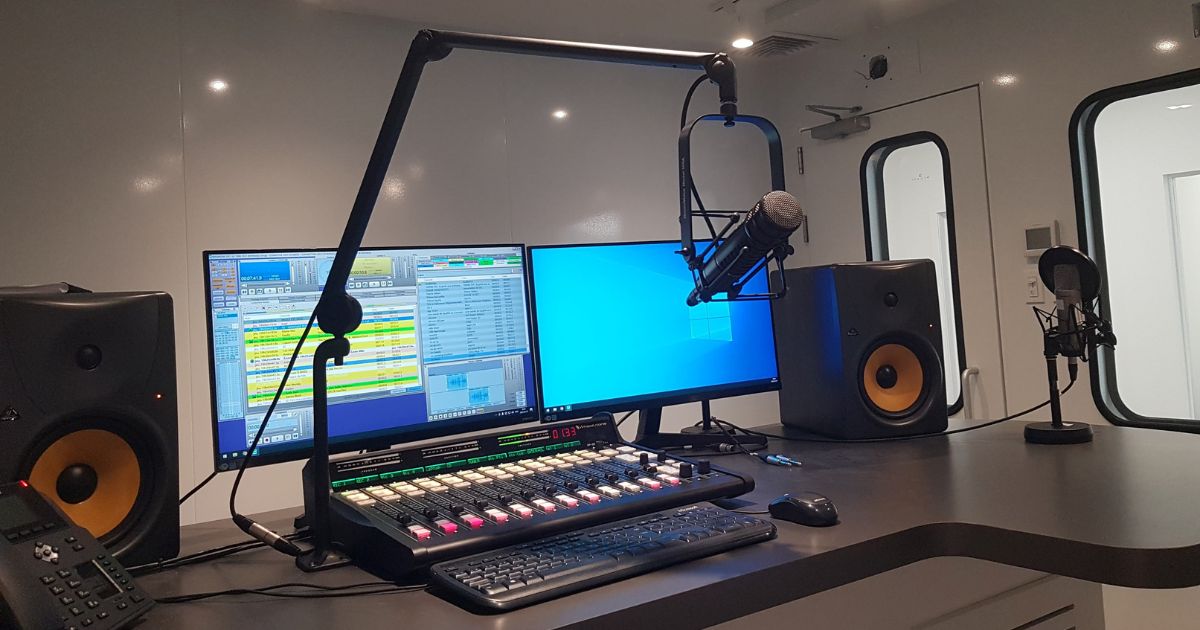This image depicts a detailed computer setup in a white-walled music studio. The brown L-shaped desk hosts an array of equipment, including two computer monitors—one displaying a blue screen and the other running a program—flanked by black speakers with orange accents. In front of the monitors are a black keyboard and mouse, alongside a sound mixer with various adjustable knobs. A prominent microphone, mounted on a pole, hangs in front of the monitors, accompanied by another microphone with a pop filter on the right side. Additional items on the desk include a black and yellow telephone in the left corner. The room features white walls with reflections from overhead lights, a door and two windows located on the right side, emphasizing the studio’s sound isolation for recording purposes.